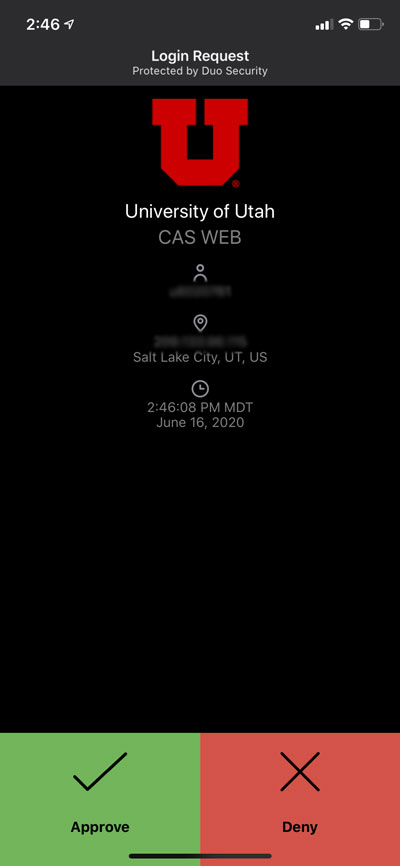A screenshot from an Android phone displays a University of Utah login request, secured by Duo Security. Dominating the top of the screen is the University of Utah's prominent logo. Below the logo, white text reads "CAS Web" against a gray background. At the bottom of the screenshot are two notable buttons: a green "Approved" button with a check mark, and a red "Deny" button with an X. The visual captures the essence of a multi-factor authentication prompt, ensuring a secure login process for university resources.